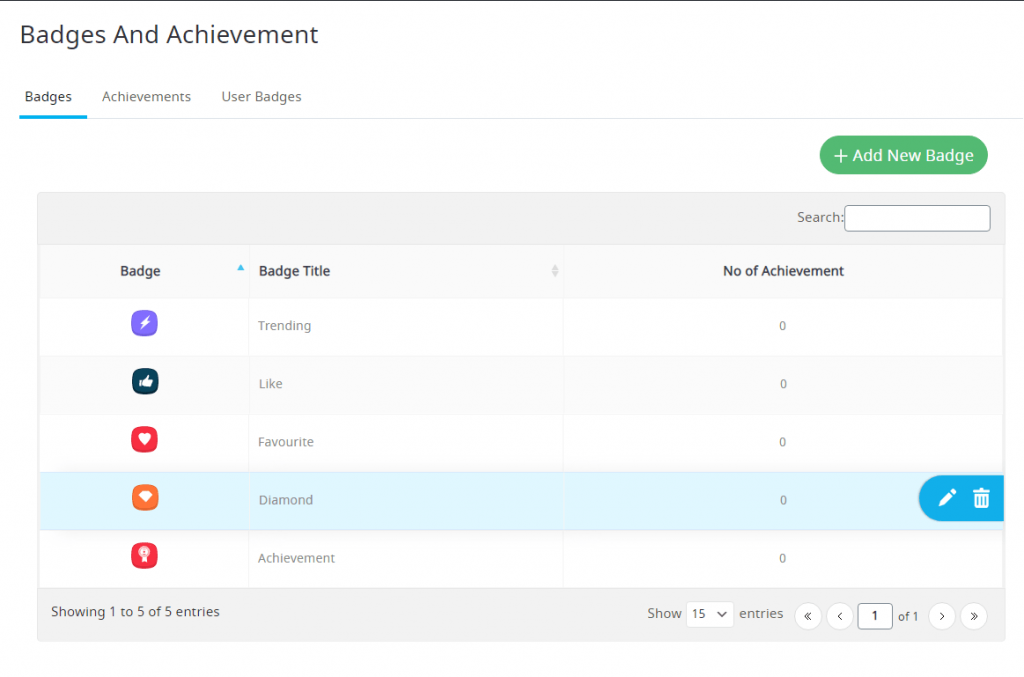The image displays a webpage designed for managing badges and achievements. At the very top, there is a thin green line, below which the text "Badges And Achievements" is prominently displayed with each word, including "And," capitalized. Underneath, the words "Badges, Achievements, User Badges" follow, with "Badges" highlighted in bold and underlined in blue.

On the right side of the page, there is a green button labeled "Add New Badge" with a plus sign next to it. Below this button, a light gray banner features a search bar with the label "Search" on its right.

The main content area alternates between light gray and white backgrounds, creating a striped effect as it lists the badges and their details. The columns are labeled "Badge," "Badge Title," and "Number of Achievements," each accompanied by small icons.

The first badge icon is purple with the label "Trending" and displays "0" achievements. The second icon is black labeled "Like," also showing "0" achievements. The third icon is red labeled "Favorite" with "0" achievements. The fourth icon, highlighted in blue, is orange and labeled "Diamond" with "0" achievements. The fifth icon is red on a white background labeled "Achievement," again with "0" achievements.

At the bottom of the content area, there is a navigation section indicating "Showing 1 to 5 of 5 entries" along with a drop-down menu for selecting the number of entries to show. Pagination controls include a left double arrow, a left arrow, a square with the number "1" indicating the current page, a right arrow, and a double right arrow.